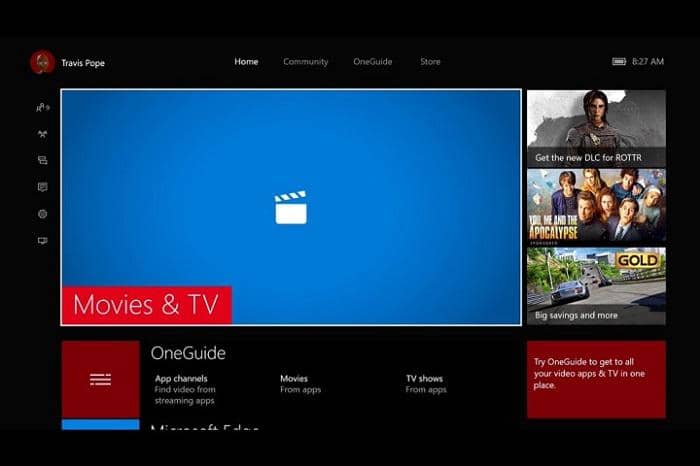Screenshot depicting the OneGuide interface of a Microsoft video system, possibly within Xbox. In the top left corner, there is a small avatar representing the user, Travis Pope. Adjacent to this, in the middle, is a horizontal menu bar with options: Home, Community, OneGuide, and Store. The top right corner displays a battery icon and the current time, 8:27 AM. On the left side of the screen, several menu icons are visible.

The primary display area shows the "Movies and TV" section, highlighted by a red background in the bottom left corner. The central portion of the screen features a blue background indicative of a loading movie clip. Directly below this, the word "OneGuide" appears, accompanied by a red square to its left. This section further details "App Channels," offering options to find videos from streaming apps, movies from apps, and TV shows from apps. In the right-hand segment of the screen, emphasized once again with a red background, is a promotional message encouraging users to try OneGuide for consolidating all their video apps and TV into one convenient platform.